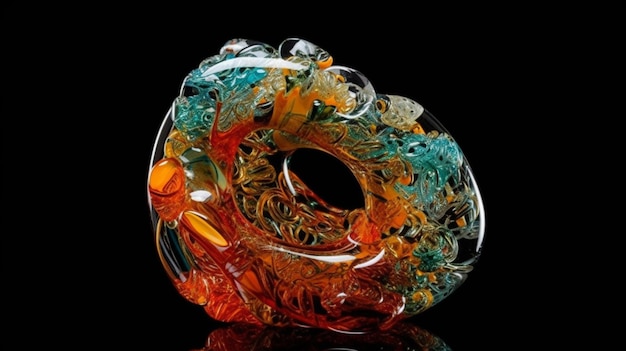On a solid jet black background, there is an intricate 3D glass object prominently displayed in the center of the image. This captivating piece appears to be handmade from blown glass, forming an oval or donut-like shape with a hole in the middle. The glass ring exhibits a mesmerizing blend of colors swirling and melting together, including blue, green, clear, red, and orange hues. This artistic fusion creates the appearance of encased elements, contributing to its decorative appeal.

Examined further, the glass object reveals a possible head-like shape at the bottom, suggestive of a dragon or similar mythical creature, predominantly in orange. Blue elements resembling flowers can be seen to the right. At the top, two fish heads are discernible: one with black eyes and brown scales, the other exhibiting black and orange tones. On the left side of the ring, there are more green glass elements and an orange blob that possibly features an eye with a black band. Enhancing its intricate design, the top part of the glass ring includes suction cups.

The glass object is flattened at the bottom, allowing it to stand upright, thus presenting a detailed and intriguing display that draws in and captivates the viewer's eye.